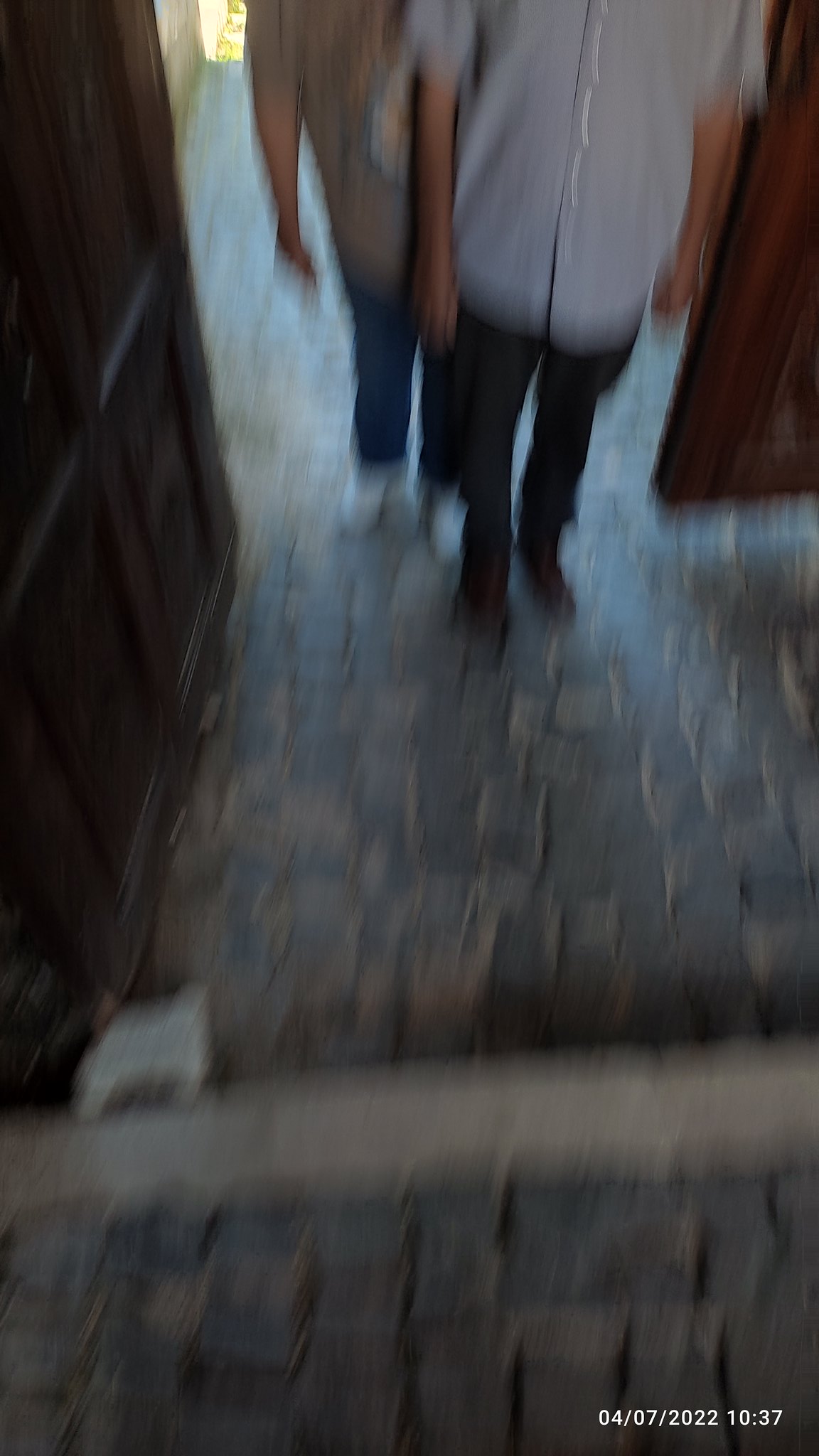In this vertically-oriented, blurred photograph, the scene is dark and colored, with the main focus being a stone walkway. At the center rear of the image, you can see two human figures standing one behind the other. The figure in front is dressed in dark pants and a short-sleeved, light-colored button-down shirt, with their arms hanging naturally by their sides. The person behind them is also wearing dark pants paired with white shoes and a short-sleeved shirt, and their arms are similarly positioned at their sides. Both figures seem to be captured in motion, possibly walking through a darkened doorway that flanks them on either side. The lower right corner of the photograph displays a timestamp in white text, reading the date "04-07-2022" and the time "10:37". The overall composition, combined with the blur and lighting, gives the image a somewhat obscure and mysterious atmosphere.